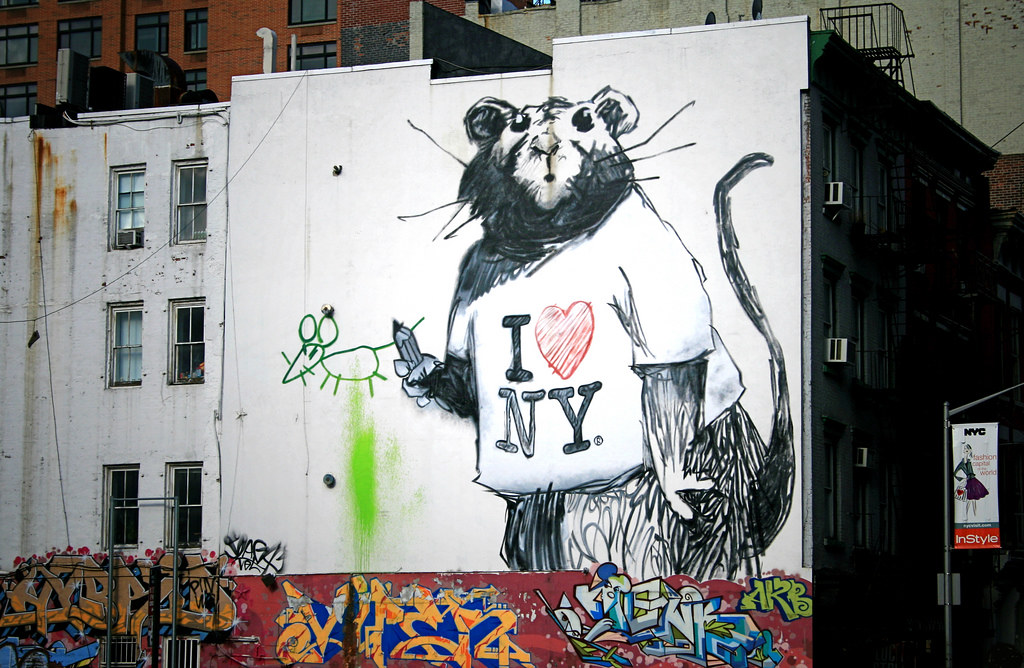The image captures a scene in New York City featuring vivid graffiti on the side of a rundown building. Dominating the wall is a large, intentionally painted, graffiti-style rat wearing a white "I ♥ NY" T-shirt, with the heart rendered in a pinkish hue. The plump rat, standing upright with a surprised expression and pronounced whiskers, holds a pencil in its right hand. Next to it, the rat has sketched a small, childlike drawing of another rat, accompanied by a green splotch beneath it. 

The building's facade, which appears to be brick, is partially covered by what seems like a smoother board for the graffiti artwork. Surrounding the main mural are various colorful tags in shades of blue, green, teal, yellow, and burgundy, suggesting a mix of different graffiti artists' contributions. 

Adjacent to this building, there is a post with a poster declaring "Fashion Capital of the World" in stylish text, featuring an image of a chic woman. This further anchors the setting as New York City, complementing the urban and creative vibe of the scene. The adjacent white building, visible to the left, has six windows spread across three floors, adding to the backdrop of this eclectic urban tableau.